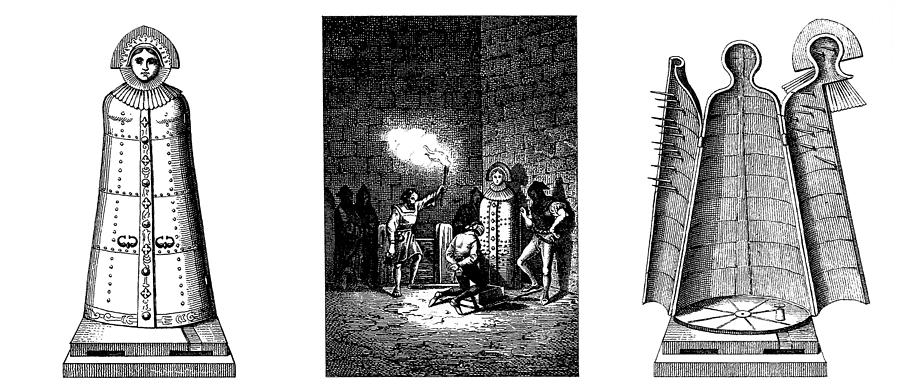The image is a detailed triptych illustration of a medieval torture device known as the Iron Maiden. In the left panel, the Iron Maiden is depicted as a statue or sculpture resembling a woman, complete with a headband, a collar around the neck, and a heavy, riveted metal coat featuring a row of crosses down the front. The figure is standing or seated on two square bases, though their material is unclear. This drawing is black and white, consistent with the pencil-like or digital illustration style used throughout.

The center panel presents a dramatic scene showing two men preparing to use the Iron Maiden on a third man, who is kneeling and blindfolded with his hands apparently handcuffed behind his back. The man on the left holds a torch, illuminating the scene, while the man on the right appears ready to open the Iron Maiden. Additionally, there are silhouettes of bystanders observing the act, adding to the tension and authenticity of this medieval scenario.

The right panel reveals the interior of the Iron Maiden, where the device is shown open to expose the menacing spikes lining its head and torso sections. This stark depiction emphasizes the brutal function of the apparatus, designed to stab and impale anyone placed inside when it is closed.